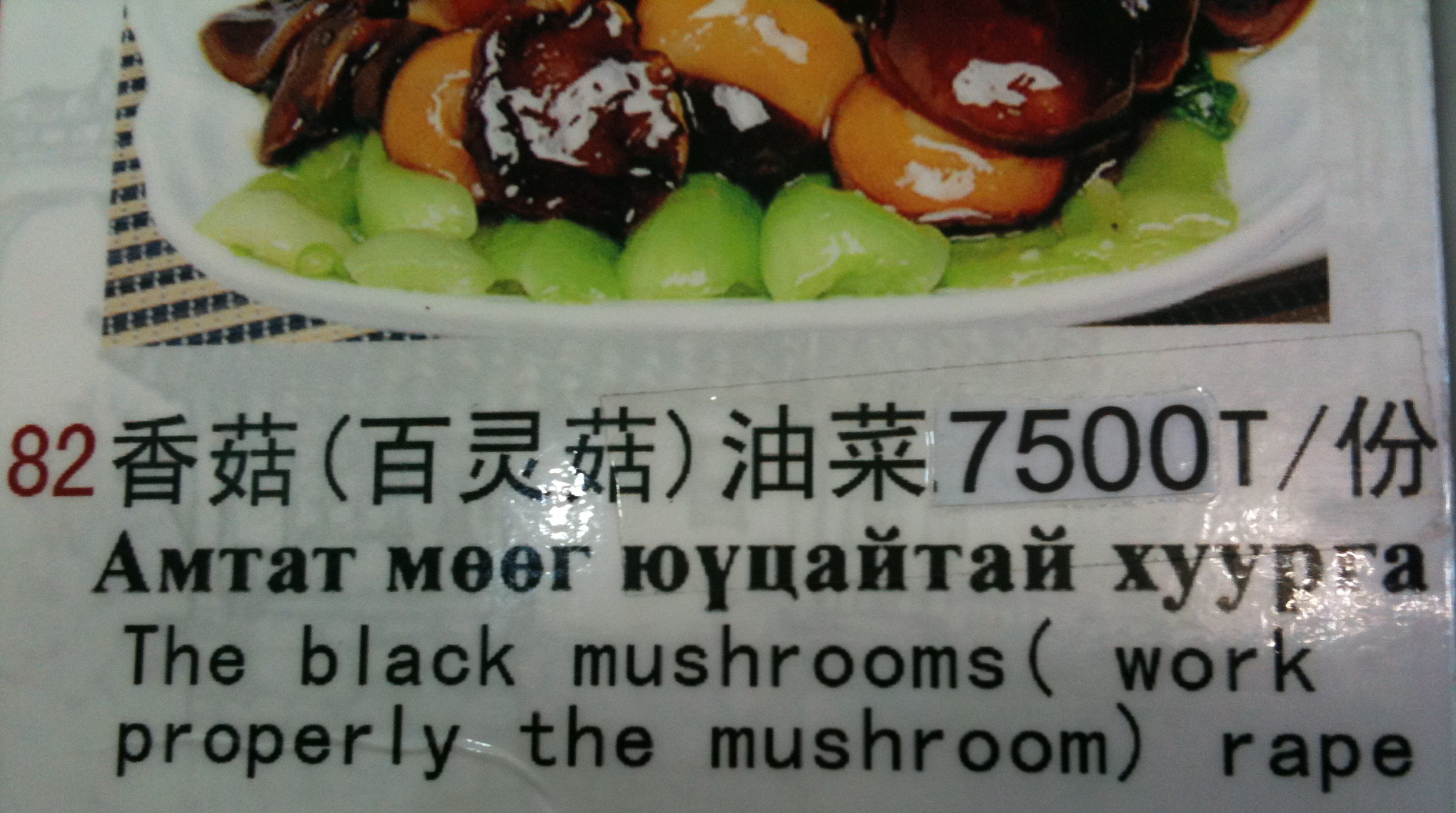This image appears to be a glossy, laminated section of a Chinese menu featuring a dish on a white plate. The dish comprises a visually appealing mix of foods: green vegetables, possibly bok choy or a green sauce resembling grapes; peach-colored glazed items, which could be meat or fruit like peaches; and mushrooms. The label includes several text elements in different languages. At the top, there is Chinese verbiage flanked by the number 82 in red. This is followed by a translation in English that reads "The black mushrooms work properly," along with some nonsensical or incorrectly translated phrases like "the mushroom rape." The entire label is set against a white background, with the text primarily in black.